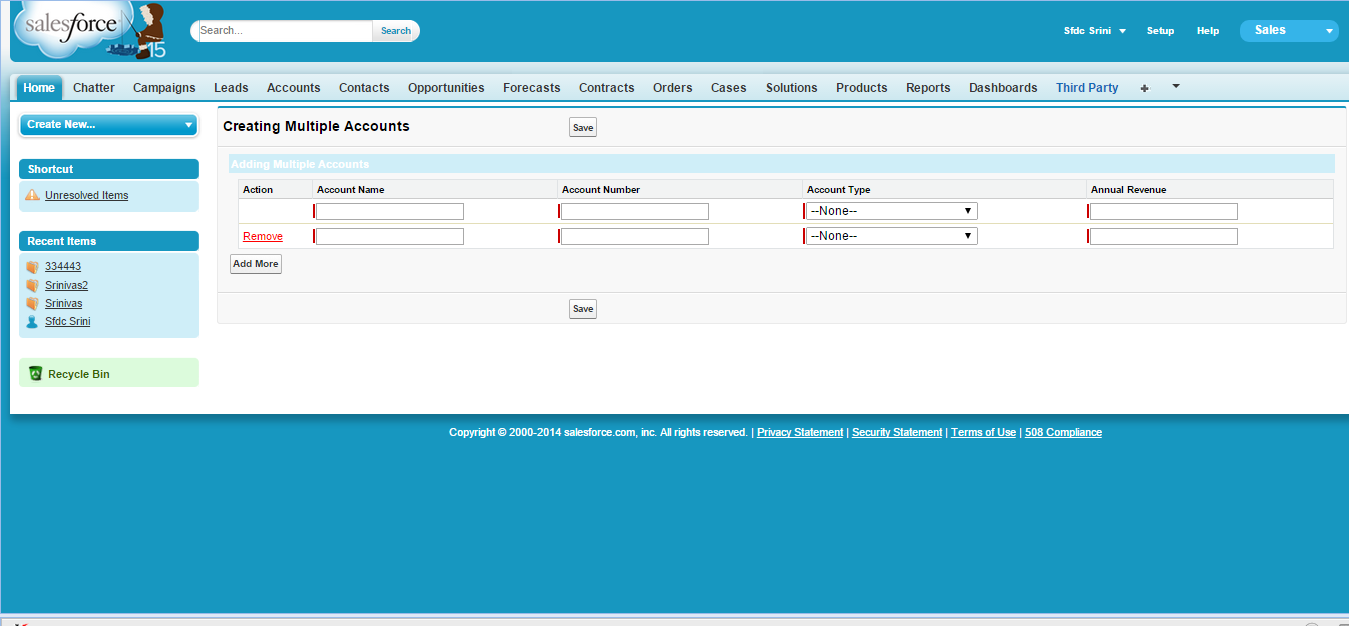The image depicts a detailed webpage interface of Salesforce. In the top left corner, the Salesforce logo is prominently displayed. To the right of the logo, there's an illustration of a person standing next to a cloud, symbolizing cloud services. Adjacent to this is a search bar, allowing users to quickly find necessary information.

In the upper-right corner, there's a dropdown menu labeled "Sales." Below this menu, a navigation list is arranged vertically, including options such as Home, Chatter, Campaign, Leads, Account, Contact, Opportunities, Forecast, Contract, Orders, Cases, Solution, Product, Report, and Dashboard.

A blue section labeled "Third Party" is featured prominently. Below this, there is a section titled "Create Multiple Accounts" which includes an actionable box labeled "Action." Adjacent columns are titled "Account Name," "Account Number," and "Account Type," which features a dropdown menu for selection. There is a "Save" button to finalize entries.

The main content area has a white background, transitioning to a light blue background towards the bottom of the page. The overall layout is organized and designed for efficient user interaction within the Salesforce platform.